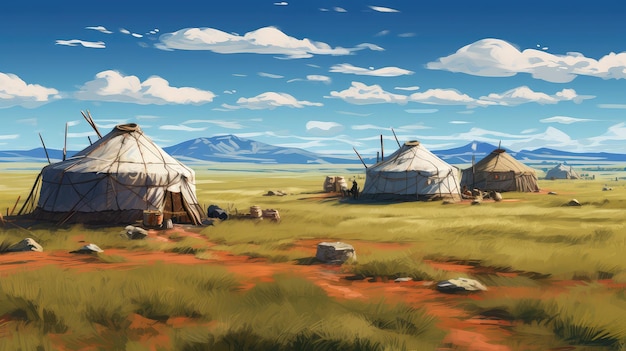This illustration depicts an expansive grassland scene under a clear blue sky dotted with fluffy cumulus clouds. Dominating the landscape are three large indigenous-style teepee tents, characterized by their cylindrical bases and conical tops. Two of these tents are white, while the one set farther back towards the right edge is brown. The ground is a patchwork of greenery interspersed with dirt and rocks, creating a rugged prairie ambience. The tents are set spaciously apart on the deserted land, with no people or supplies visible, emphasizing the isolation of the setting. In the background, majestic blue mountains rise up, adding depth and a sense of grandeur to the scene.